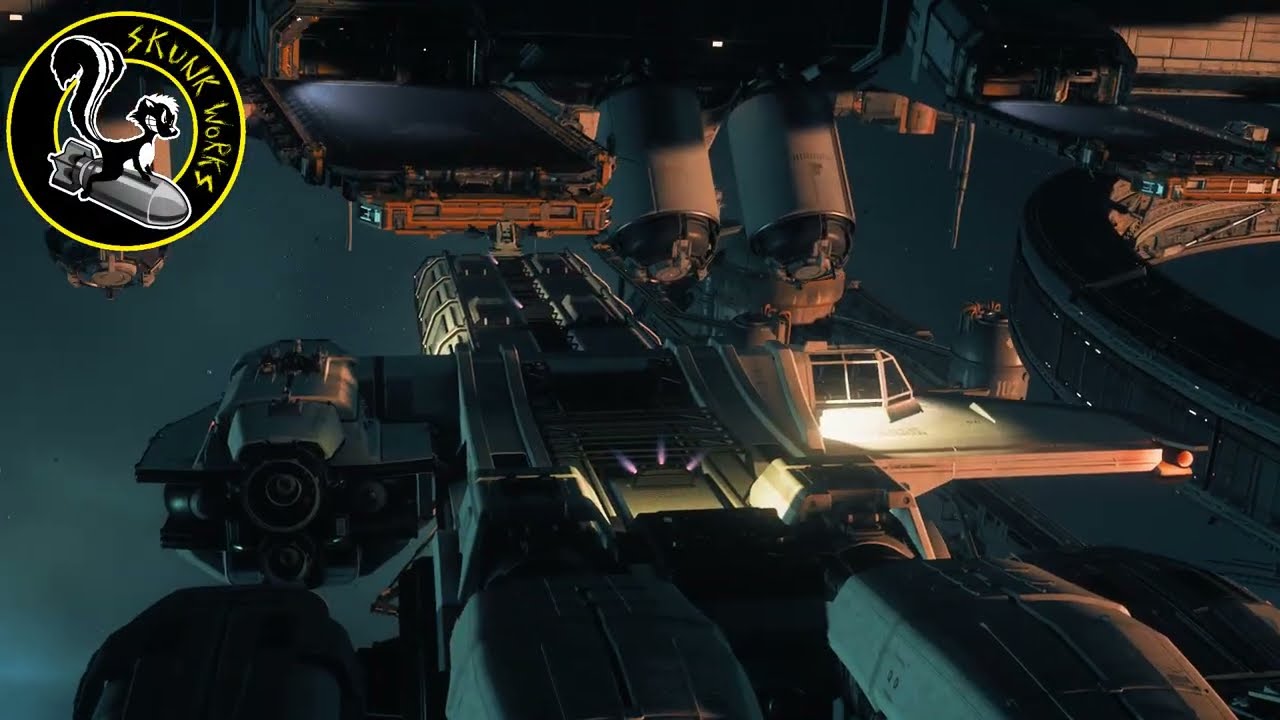The image depicts a computer-generated scene primarily showcasing a spaceship against the backdrop of outer space. In the upper left-hand corner, there is a prominent "Skunk Works" logo featuring a black and white skunk on a grey rocket with yellow text. The main focus is the spaceship itself, characterized by a combination of metallic silvers and blacks, with a detailed, multi-level structure. The front of the ship features a rectangular section with a glass window, which then widens through the center and narrows slightly towards the back, incorporating cylindrical engines. Adjacent to this main body is a large circular structure with an empty center space, and other smaller platforms extending out from the ship, one of which resembles a landing bay. The scene is illuminated by a soft orangey light, enhancing the intricate details of the mechanical components, while the dark teal-blue space background, dotted with faint white stars, emphasizes the vessel's presence in the cosmos. The image conveys a sense of advanced technology and exploration, possibly hinting at a futuristic space mission.